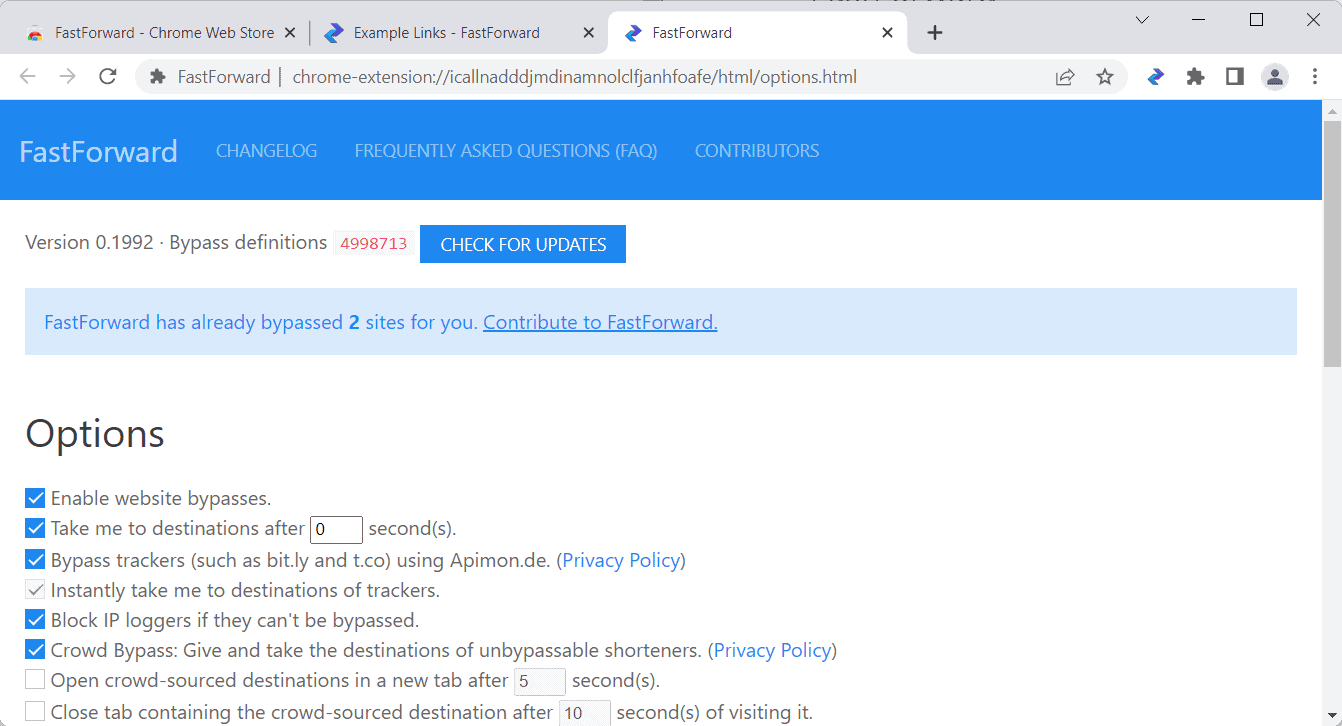A user is currently browsing multiple tabs in Google Chrome, prominently featuring a webpage for a Chrome extension called "Fast Forward." The extension's interface displays a light blue background with slightly faded white text, overlaying a white section with black text.

Details on the page include:
- The "Fast Forward" logo and sections: Change Log, Frequently Asked Questions, Contributions, and Contributors.
- Version number: 0.1992, and a red notification with the ID 4998713.
- A prompt to "Check for Updates."

Highlighted are functionalities of the extension:
- A statement reads, "Fast Forward, I have bypassed two sites for you."
- An encouragement to "Contribute to Fast Forward."
- An options panel with several checkboxes:
  - "Enable Website Bypasses" (checked in blue)
  - "Take me to stations after zero seconds"
  - Bypass trackers like Bitly and Tico using appanon.d
  - An option to "Instantly take me to destination trackers" (white check)
  - "Block IP loggers if they can't be bypassed"
  - "Crowd bypass" with choices like "Give me take destination unbypassed"
  - Settings for handling shorteners and crowdsourced destinations, including options to:
    - Open the crowdsourced destination in a new tab after five seconds
    - Close the tab containing the crowdsourced destination after ten seconds of visiting.

Additional webpages open include the Fast Forward Chrome Web Store and example links for the extension.

Overall, the user seems engaged in configuring the various bypass and security features of the "Fast Forward" extension to enhance their browsing experience.